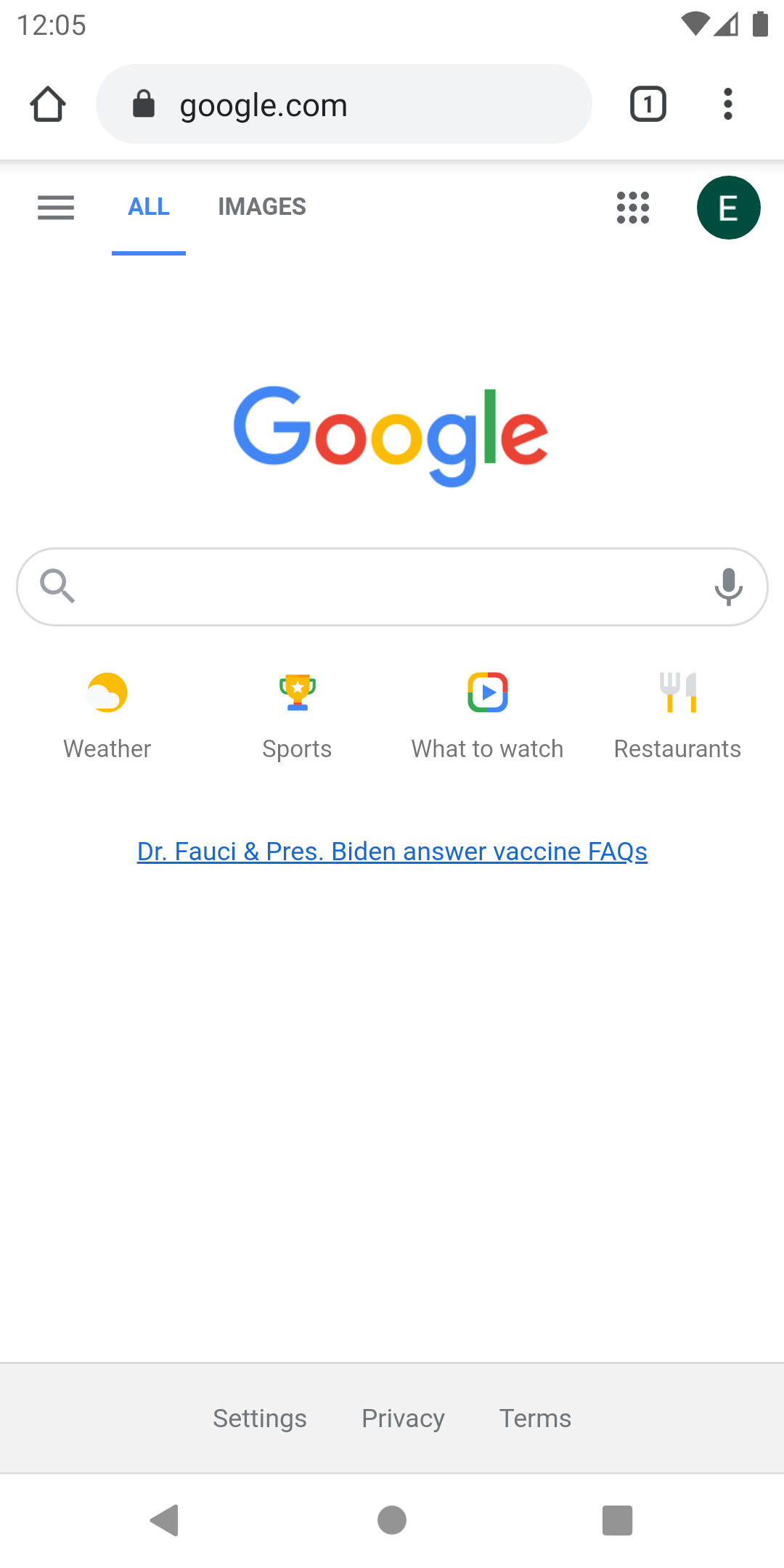The image is a detailed screenshot of a smartphone displaying the Google search page. In the status bar at the top, the time is shown as 12:05 on the left, while the right side displays full network signal bars and a fully charged battery icon. The main content area starts with the Google search bar, housed within a gray pill-shaped box labeled "Google.com" accompanied by a padlock icon indicating a secure connection. To the left of the search bar, there is a home icon, while the right side shows a number "1" in a square and a three-dot menu.

Below the search bar, a navigation bar contains three horizontal black lines for the menu, a blue underlined "All" option, and additional tabs for "Images." Towards the right, there is an icon with three rows of three dots and an "E" in a black circle. The familiar Google logo, featuring a capital "G" in blue, a small "o" in red, a small "o" in yellow, a lowercase "g" in blue, an "l" in green, and an "e" in red, is prominently displayed. Immediately below this logo is the main search bar, including a magnifying glass icon on the left and a microphone icon on the right.

Directly beneath the search bar are several quick-access options: "Weather" with a sun and cloud icon, "Sports" with a yellow trophy, "What to Watch" featuring a TV outline with a play arrow, and "Restaurants" symbolized by a fork and knife. An underlined blue link reads, "Dr. Fauci and Prez Biden answer vaccine FAQs." At the bottom, there is a gray footer bar with "Settings," "Privacy," and "Terms" links. Finally, three icons in gray are displayed: a left-facing arrow, a circle, and a square.